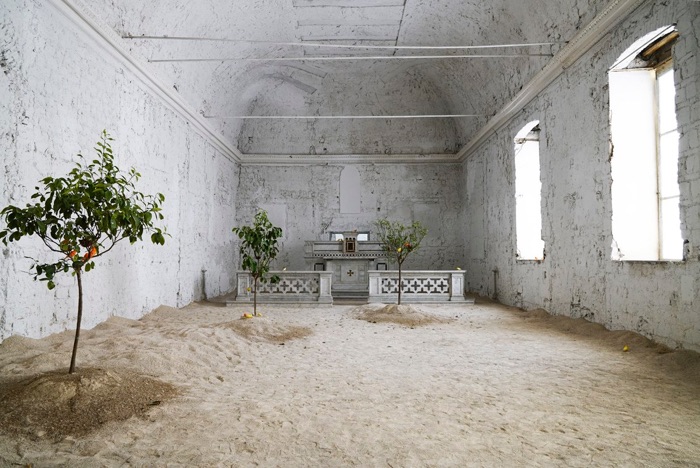This image captures what appears to be an abandoned and possibly repurposed church building, depicted in strikingly realistic detail. The building, predominantly whitewashed, features painted over stone or brick walls and an arched ceiling that resembles half of a cylinder. The paint on the walls is noticeably chipping, adding to the aged atmosphere of the interior.

The floor is entirely covered with soil, giving an unusual contrast to the indoor setting. Planted within this soil are three small fruit trees, likely an orange tree, a lemon tree, and a grapefruit tree, each standing about seven to eight feet tall. Despite their youth, one tree appears to bear peaches, and there are two pieces of fruit lying on the ground.

The room is well-lit by natural sunlight streaming through two large carved-out windows on the right side. The windows highlight thin metal beams or braces stretching across the ceiling, possibly serving as supports for the structure. In the center of the photo, where one might expect a pulpit, stands an altar with a white mantle featuring a grid-style design. This area is flanked by a small fence or railing, about two feet tall, adding to the sense of a sacred space.

Overall, the image portrays a space that blends the sacred with the natural, the ancient with the repurposed, creating a unique and thought-provoking scene.